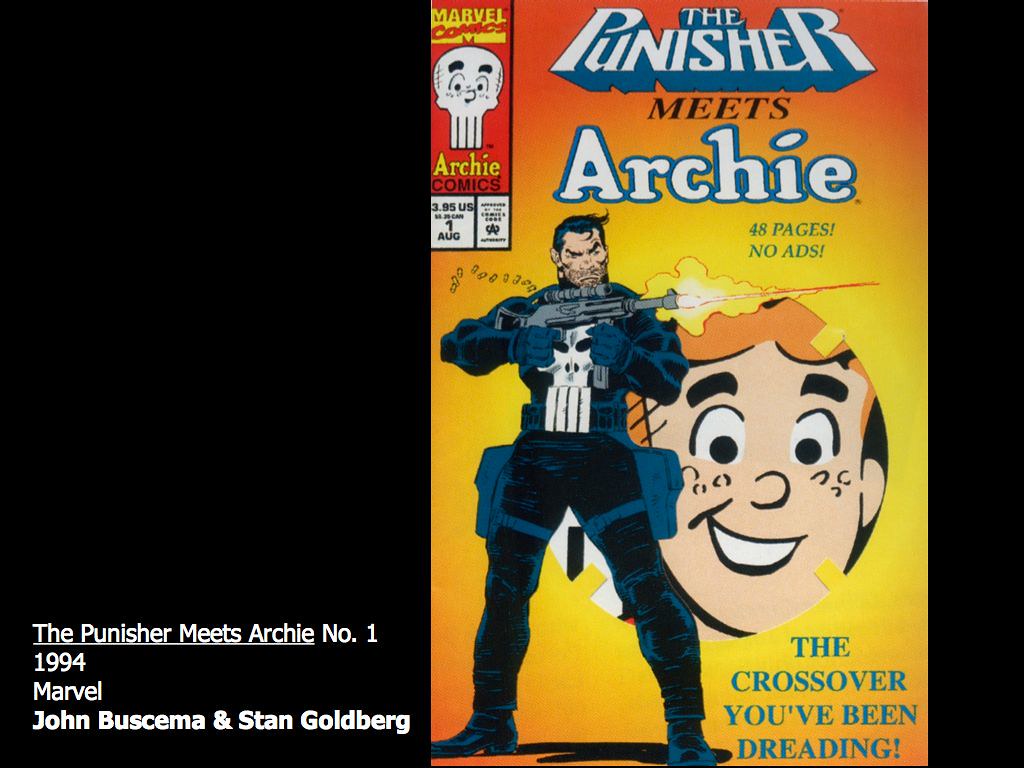This image appears to be a framed comic book cover with significant details and descriptions. The cover, encased in a black frame, prominently displays the title "The Punisher meets Archie No. 1, 1994, Marvel," attributed to John Buscema and Stan Goldberg. In the bottom left-hand corner of the frame, this identifying information is clearly written in white letters. The comic book cover itself features a dark orange top that transitions into a gold background, with a muscular, grim-looking character known as The Punisher, dressed in a black outfit with a white skull on his chest, holding and firing a flaming machine gun. The top left corner of the cover has a red square with "Marvel Comics" and "Archie Comics" logos, and the price "$3.95 US" alongside the date "1 August" displayed in a white box below. The title "The Punisher meets Archie" is written in large, distinct letters and declares "48 pages, no ads" in the top third of the cover. Behind The Punisher, a circle inset features a smiling, simplistic cartoon face of Archie. The bottom right-hand corner of the cover ominously states, "The crossover you've been dreading!"